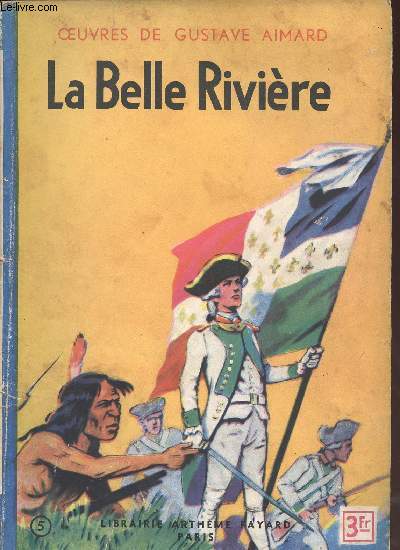The image is a detailed scan of what appears to be a French book cover with a predominantly yellow-orange background, possibly titled "La Belle Riviere." In black, bold text, the title is prominently displayed across the center of the cover. At the very top, in smaller red text, reads "OEUVRES DE GUSTAVE AIMARD." The cover features an elaborate illustration with colonial-era military and native figures. The central figure is a soldier dressed in a white uniform with green trim, wearing a black hat with gold accents, holding a large flag. This flag includes a white cross adorned with golden fleurs-de-lis and four quadrants colored blue, red, orange, and green. Surrounding this central soldier are two other military men, one shouldering a rifle, both in similar uniforms and tricorn hats. In the bottom left corner of the illustration, a Native American man with a feather in his hair is depicted crouching and pointing, seemingly amidst grass. Additional text in black at the bottom of the cover reads "Librairie Artime Hayard Paris," and there is a price tag in the bottom right corner indicating "three francs." A black circled number five appears in the bottom left. The top left corner features a watermark or website address, "le-livre.com."